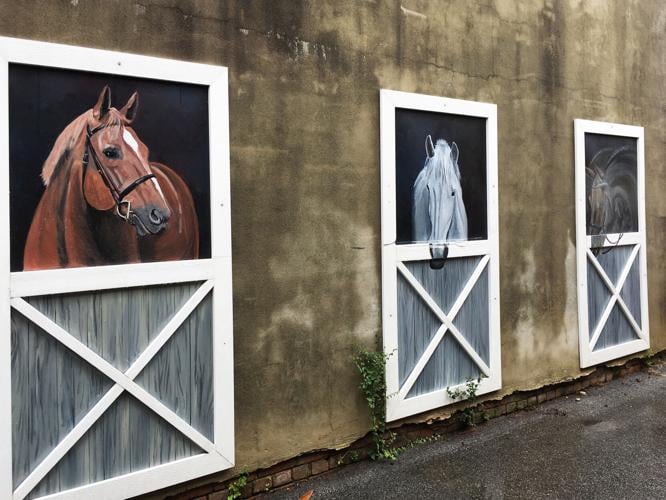The image captures a vivid mural painted on the side of an aged concrete building with a red brick base and climbing vines. The mural features a lifelike depiction of three horse stables with white barn doors, each showcasing a different horse gazing out onto the street. The horses are painted with a remarkable three-dimensional effect, giving the illusion that they are peering out from actual stalls. On the left, a brown horse with a white spot between its eyes and a bridle stands out. The center stall houses a solid white horse with a touch of black on its nose, also looking out with keen interest. On the right, a darker brown horse, also in a bridle, peers over the stable window. The scene is set in daylight, and the mural's detail and depth bring the horses to life, making them appear almost real to passersby.